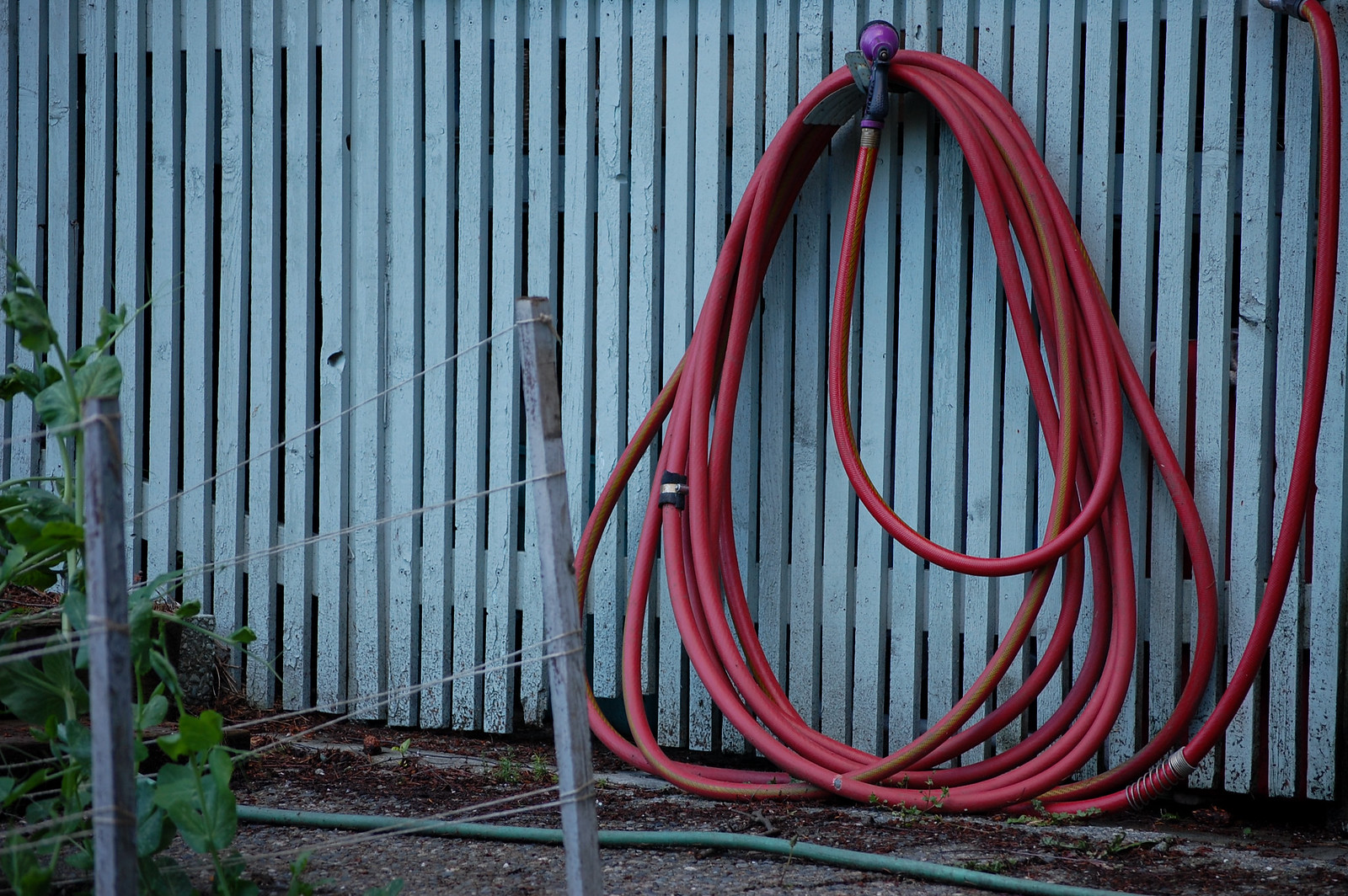This image showcases a light baby blue wooden fence adorned with a red hose that descends from the right, making wide loops around a metal bracket on the fence. The hose ends with a purple nozzled sprayer, accented by a black handle, clipped at the top of the loops. Below, a green hose lies across a dirt path, accompanied by a smattering of green foliage in the bottom left corner. Additionally, there is a gray fence post wrapped with twine, contributing to the rustic setting. The scene suggests a garden environment, possibly just maintained, as evidenced by trimmed weeds and well-placed elements.